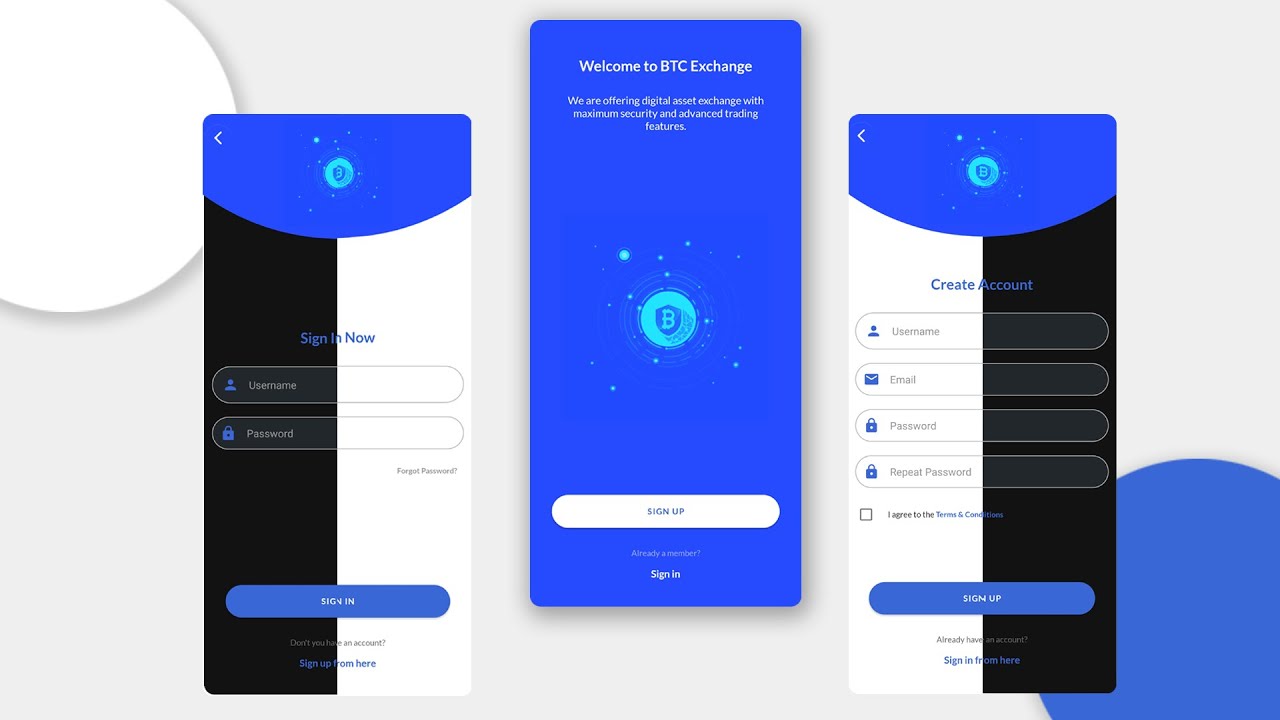This is a detailed screenshot of a website that appears to guide users on how to sign in to an app. The background in the upper left corner is gray, contrasting with a portion of a white circle in the lower right, intersected by a fragment of a blue circle. At the center of the image, there are three small graphics representing smartphone screens. These are quite detailed although small in size.

The first graphic, on the left, demonstrates the sign-in process with text fields labeled "Username" and "Password" along with a "Sign In Now" button. The central graphic welcomes users to "BTC Exchange" with a message that reads: "Welcome to BTC Exchange. We are offering digital asset exchange with maximum security and trading fortunes." This section is designed in blue, featuring a white circular logo with a "B" in the center. The graphic on the right shows the "Create Account" screen, displaying various fields required for account creation. Overall, the screenshot serves as a visual tutorial on signing in to and creating an account on the app.